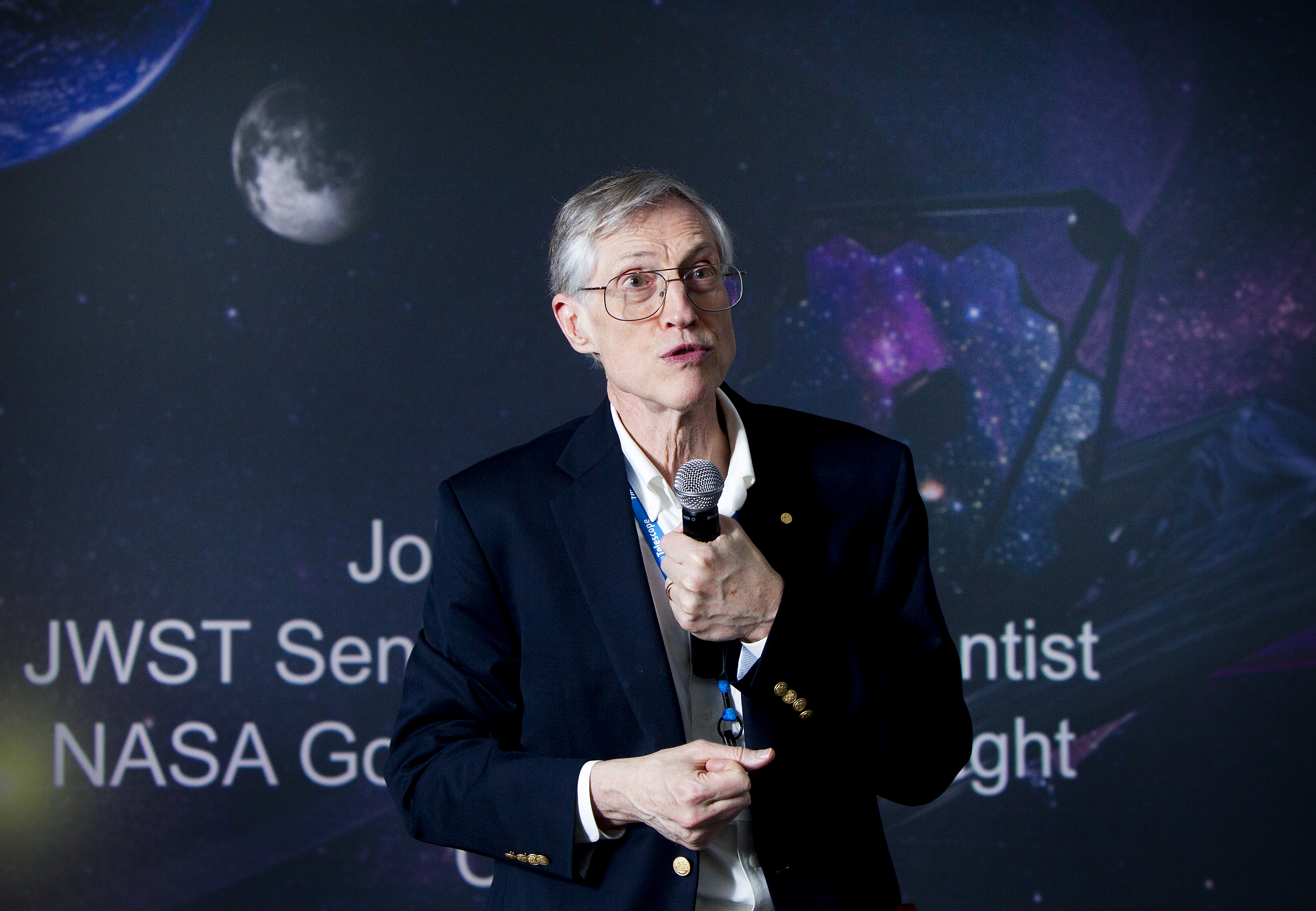The photograph captures a detailed scene of an older gentleman, visible from the waist up, engaging in a conversation. He wears a blue business coat adorned with gold buttons over a white button-up shirt, with the top two buttons casually undone. A blue lanyard hangs around his neck. His face is characterized by large, wire-framed, rectangular glasses and grey hair, with subtle signs of age, such as a wrinkled neck and veins visible on his hands. His mouth is partly open, suggesting he is in mid-conversation, while he holds a black-handled microphone with a silver top near his neck. 

In the background, a vivid night sky adorned with stars is visible, along with partial views of Earth and the moon in the upper-left corner. Both celestial bodies contribute to the backdrop's cosmic feel. White lettering, partially obscured by the man's body, spells out "J-O" followed by "J-W-S-T," and "N-A-S-A." The scene suggests a formal or scientific setting, potentially relating to a NASA event or announcement.